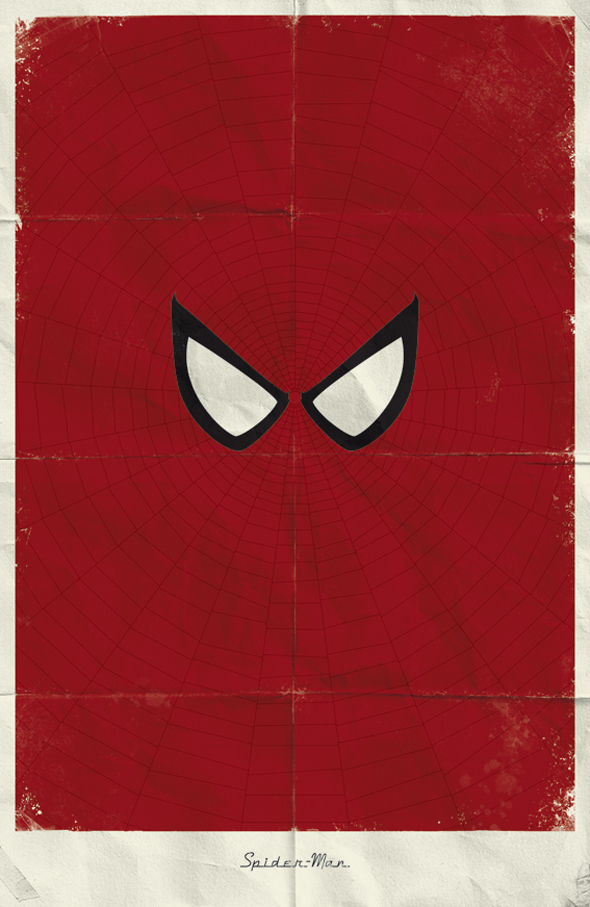The image depicts a worn, rectangular paper poster with multiple visible creases indicating it had been folded into squares. The poster has a thin white border and a faded red background, particularly along the fold lines. At the bottom, in bold black letters, it reads "Spider-Man." Dominating the poster are two distinct, teardrop-shaped eyes lined in black with white centers, resembling the iconic eyes on Spider-Man's mask. These eyes point towards the upper corners of the poster. Radiating outward from the eyes is a spider web pattern, delicately branching out in light red and black lines, accentuating the Spider-Man theme.